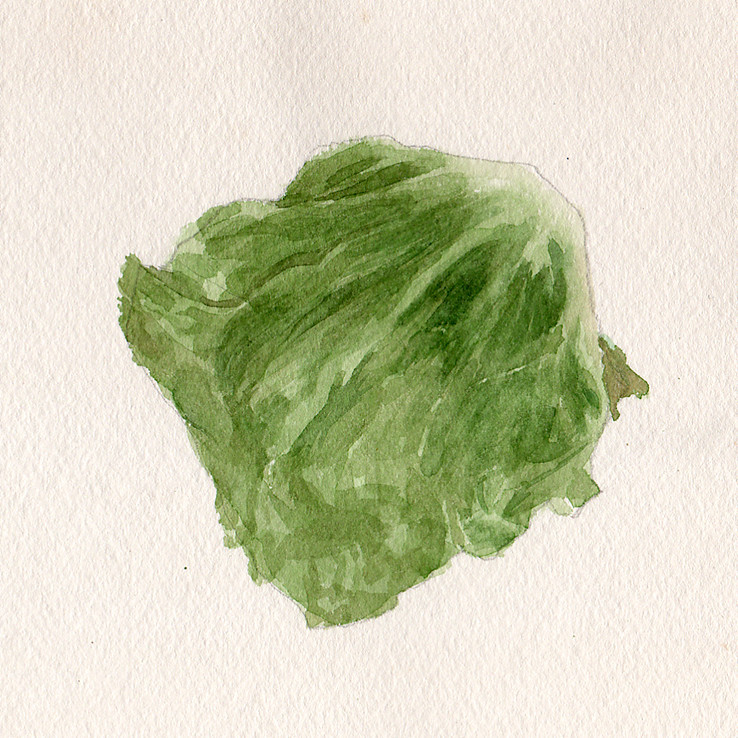This image showcases a detailed watercolor painting of a single, slightly wilted iceberg lettuce leaf. The painting was first sketched in pencil, evident from the faint outlines that frame the subject, and then filled in with varying shades of green watercolor. The leaf is vaguely square-shaped and positioned at an angle, with the top right being a light green, almost whitish hue, gradually darkening as it moves down to the left. The painting is done on fancy, textured watercolor paper, giving it a distinct artistic feel. The leaf appears somewhat slimy, as though it has been sitting out for a while, contributing to its wilted appearance. There is no text or signature on the piece, and the setting is indoors, indicating that the artist might have aimed to study the leaf closely or perhaps comment on its condition. The overall mood suggests a careful observation of the lettuce, highlighting both its form and texture meticulously.